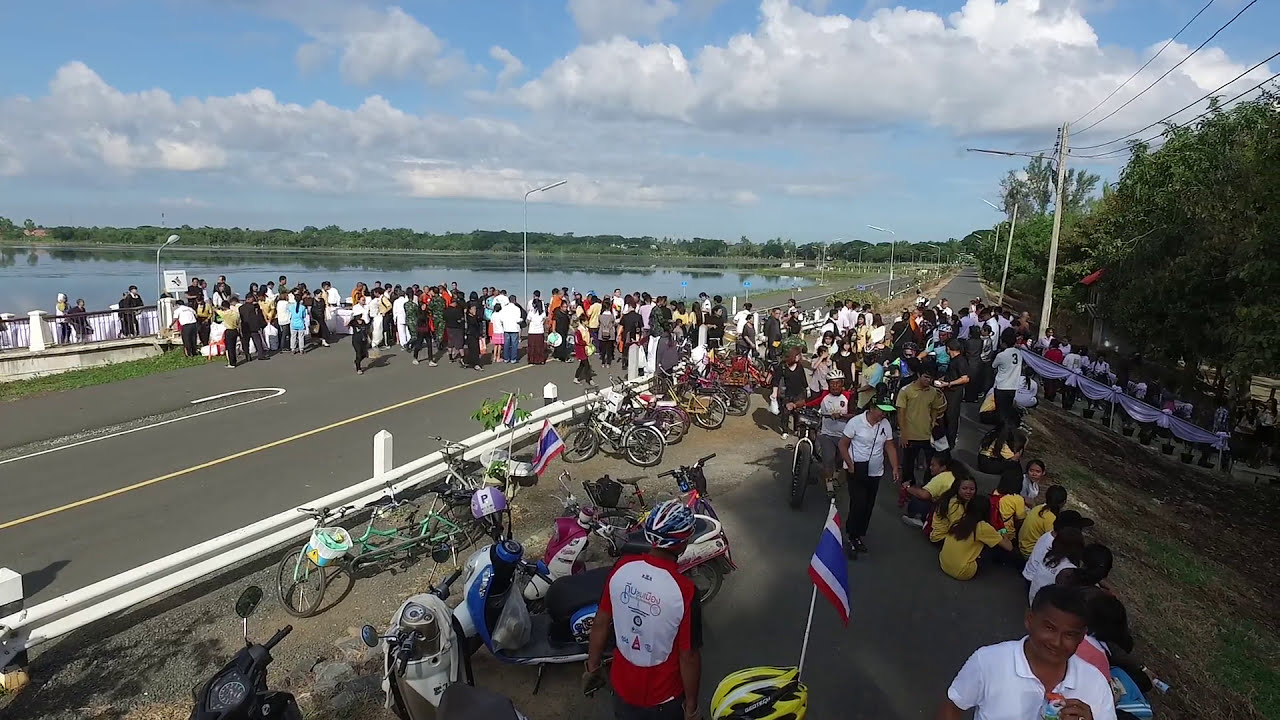A large crowd of people with dark complexions has gathered on a sunny day with a notably blue sky scattered with cumulus clouds. The scene is set on a roadway that overlooks a body of water, possibly a lake, bordered in the background by both small and large trees and a few telephone poles with wires. People are congesting the road, effectively blocking traffic, suggesting it might be a protest or a public gathering. On the right side of the image, there are numerous bicycles and motor scooters parked along a pathway, possibly a bike trail, next to a small guardrail fence. Additionally, a flag featuring blue, white, and red stripes is visible on the right-hand side, adding a colorful detail to the assembly. The atmosphere, while clearly busy and active, is underlined by a sense of a pleasant day outdoors.